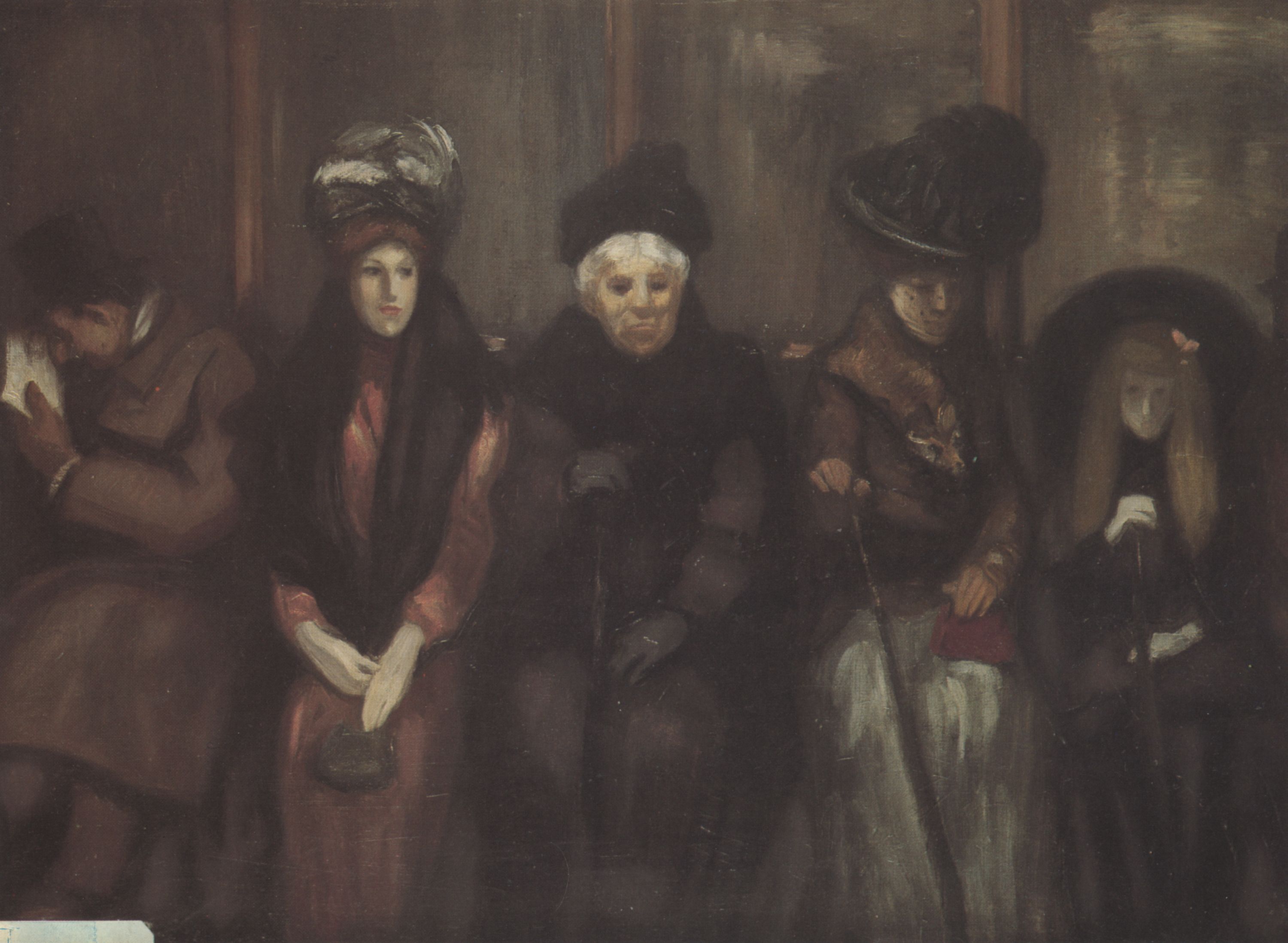The painting is a rectangular artwork, wider than it is tall, featuring a line of figures against a dark, grayish-black wall. From left to right, the scene begins with a man in a long dark gray coat, black gloves, and a black hat, sitting and hunched over, engrossed in a piece of paper. His back faces a woman in a dark pink dress with a whitish-gray hat and a dark scarf, carrying a small handbag.

In the center stands an older woman, distinguished by her white hair and a black hat, dressed in gray with a black shawl over her shoulders. She stands out, looking directly at us with an air of solemnity. To her right, another woman gazes slightly to the right, wearing a dark pink top over a dark gray dress, adorned with a faux fur collar, and holding a red purse. She too wears a dark hat, and brown gloves, and holds a cane.

On the far right stands the smallest figure, possibly a young girl with long, light-colored hair adorned with a pink or light-colored accessory. She wears a large black hat, white gloves, and a black dress. Her face is starkly white, adding a haunting quality to her appearance. All figures are dressed warmly, implying colder weather, with each donning various hats and gloves, contributing to the painting's dark and muted palette of blacks, reds, browns, and grays.